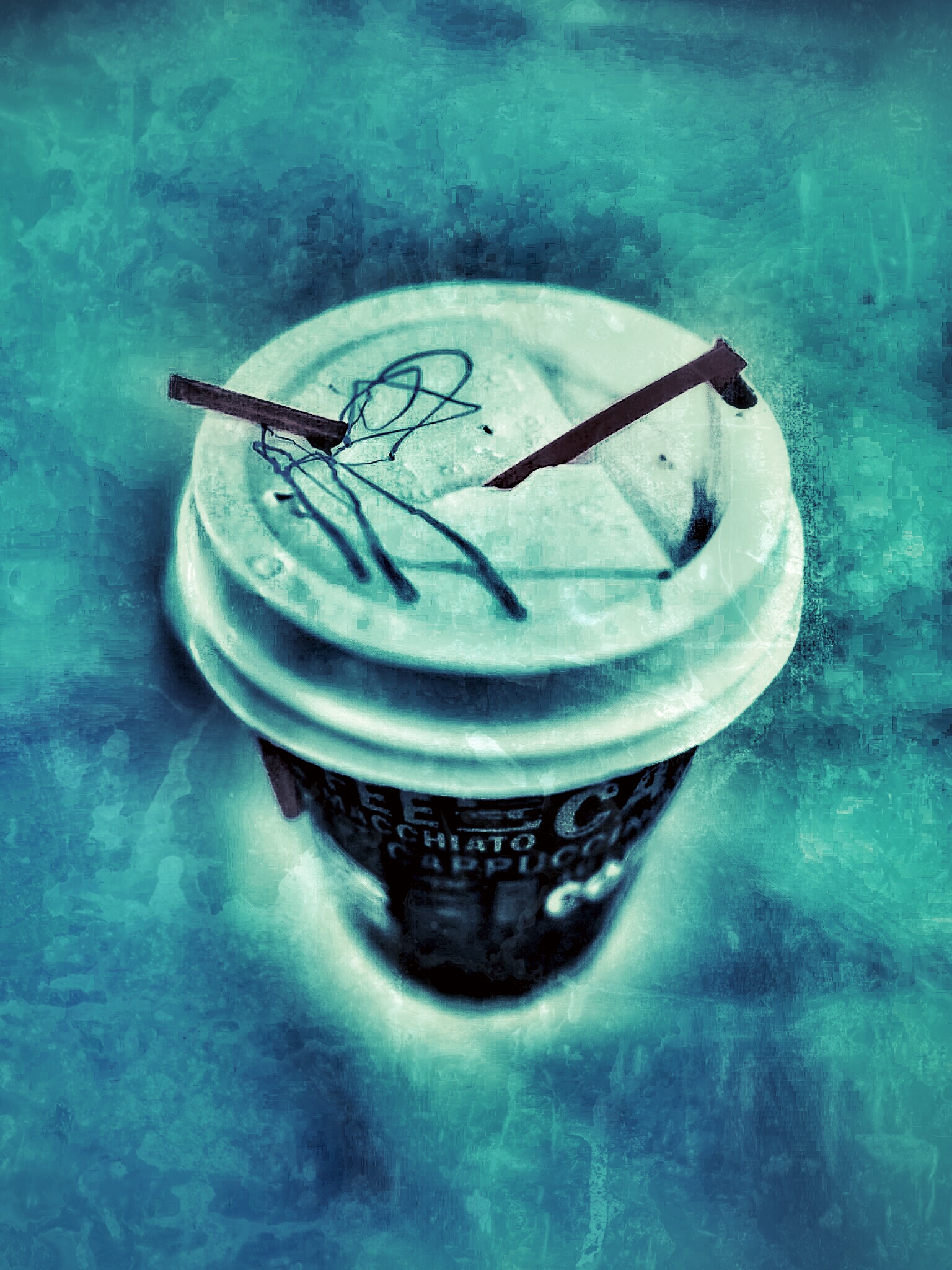The artwork depicts a surreal, vertical-oriented image featuring a dark brown or black disposable coffee cup with a white plastic lid, akin to those found in coffee shops like Starbucks. The lid is punctured by what appears to be a straw or coffee stirrer, and around it, there are multiple strings, including some dark blue ones. The cup is adorned with words such as "macchiato," "cappuccino," "coffee," and "cafe." The background is a textured mix of light and dark blues, evoking a cold, Arctic feel, reminiscent of the Aurora Borealis. The entire piece has a glowing white aura at the bottom of the cup and is executed in a somewhat abstract, splotchy style that blurs the distinction between a drawing and a filtered photograph, giving it an overall surreal and dreamlike quality.